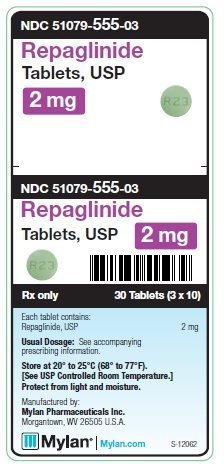The image features a detailed visual of prescription medication labeled as NDC 51079-555-03. The primary focus is a smartphone-like screen displaying the product information for "Repuglinaid Tablets USB." The key details highlighted include: 

- **Medication Name**: Repuglinaid Tablets USB
- **Dosage**: 2mg per tablet
- **Identification Code**: R23
- **Appearance**: Gray, square-shaped tablets
- **Packaging Information**: The label "RX only" indicating prescription-only status, with a total of 30 tablets, divided into 3 blister packs of 10 tablets each (3x10).
- **Manufacturer's Website**: mylan.com
- **Batch Identifier**: S-12062

The background of the image is a clean, stark white, bringing attention to the structured layout of the text and tablet imagery, ensuring clarity and focus on the medication details.